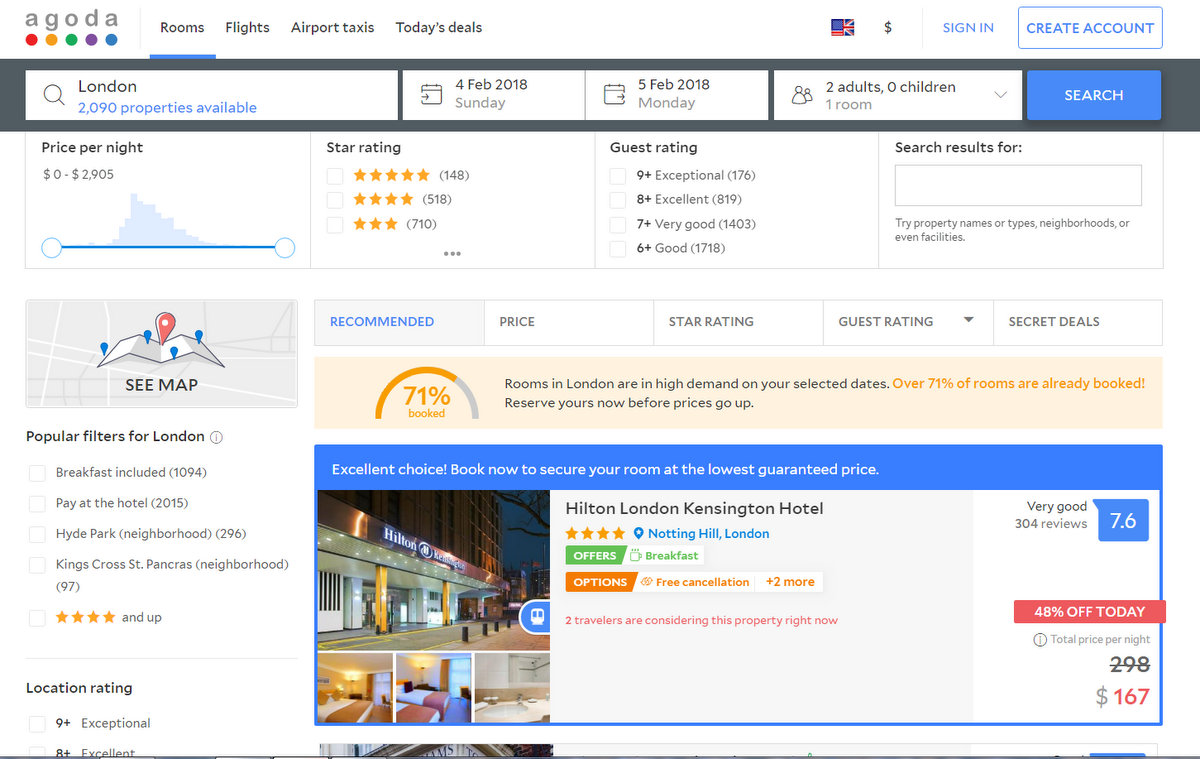This detailed caption offers a vivid description of an Agoda web page showcasing accommodation options in London:

---

The web page has a clean, white background. Positioned in the top left corner, there is a logo feature with grey text that reads "AGODA", underlined by a series of colored circles: a red circle beneath the 'A', an orange circle under the 'G', a green circle under the 'O', a purple circle under the 'D', and a blue circle under the final 'A'. Below the logo are clickable tabs labeled "Rooms" (with a blue underline), "Flights", "Airport Taxis", and "Today's Deals".

On the right-hand side of the header, there is an icon that appears to blend the British flag with another unrecognizable flag, followed by a dollar sign. Adjacent to these icons, the text "Sign In" appears in blue hyperlink format, next to a blue-bordered rectangle with blue text that reads "Create Account".

In the center of the page, there is a black bezel containing a search field marked by a magnifying glass icon. Next to the icon, the word "London" is displayed in grey. Beneath this, in blue hyperlink text, it states "2090 properties available". To the right of this search field are several rectangular icons:
1. A calendar icon showing "4th of February 2018, Sunday" with an arrow pointing to the right, followed by "5th of February 2018, Monday".
2. An icon with two silhouettes, labeled "2 adults, 0 children, 1 room".
3. A dark blue rectangle with white text saying "Search".

On the left side of the page, there is a section detailing price per night ranging from $0 to $2905, represented graphically with a fluctuating blue line. Below is a star rating filter with black text including:
- Five stars (148 reviews)
- Four stars (518 reviews)
- Three stars (710 reviews)

Further down, guest rating filters are available, each in grey rectangles:
- 9+ (Exceptional, 178 reviews)
- 8+ (Excellent, 819 reviews)
- 7+ (Very Good, 1403 reviews)
- 6+ (Good, 1718 reviews)

Towards the far right of the page, there is a search prompt, encouraging users to try searching by property names, types, neighborhoods, or even landmarks within a blank input box.

The website's sidebar on the left features a grey map section with blue and red pins, labeled "CAMP". Popular filters for London are shown in bold black text, with various selectable options:
- "Breakfast Included" (1094 properties)
- "Pay at Hotel" (215 properties)
- "Hyde Park (neighborhood)" (296 properties)
- "Kings Cross St. Pancras (neighborhood)" (97 properties)

Further down, icon representations for location ratings display:
- 9+ (Exceptional)
- 8+ (Excellent)

An orange rectangle denotes "71% booked", indicating high demand for rooms in London on the selected dates. It warns in black text, "Rooms in London are in high demand on your selected dates" and emphasizes in orange, "Over 71% of rooms have already been booked!" urging users to "Reserve yours now before prices go up."

The main section of the page showcases a specific hotel listing for the "Hilton London Kensington Hotel", rated with four stars. Nearby navigational pin icon and hyperlink text identify the location as "Notting Hill, London". Multiple labels are slanted across the hotel image:
- Green rectangle: "Offers"
- White rectangle: "Breakfast"
- Orange rectangle: "Options"
- Another label reading "Free Cancellations" and an orange note "Plus two more"

A prompt in dark blue reads, "Excellent choice! Book now to secure your room at the lowest guaranteed price." On the right, the hotel's rating is noted as "7.6 (Very Good)" from 304 reviews, with a highlighted blue square containing a pin icon.

An enticing offer is displayed within a red rectangle stating "48% Off Today", under which, in grey, a circled 'i' for information leads to text showing the original price of $298 (crossed out), with the discount bringing it down to $168.67. 

---

This enriched description provides a comprehensive and structured overview of the Agoda booking page for users.